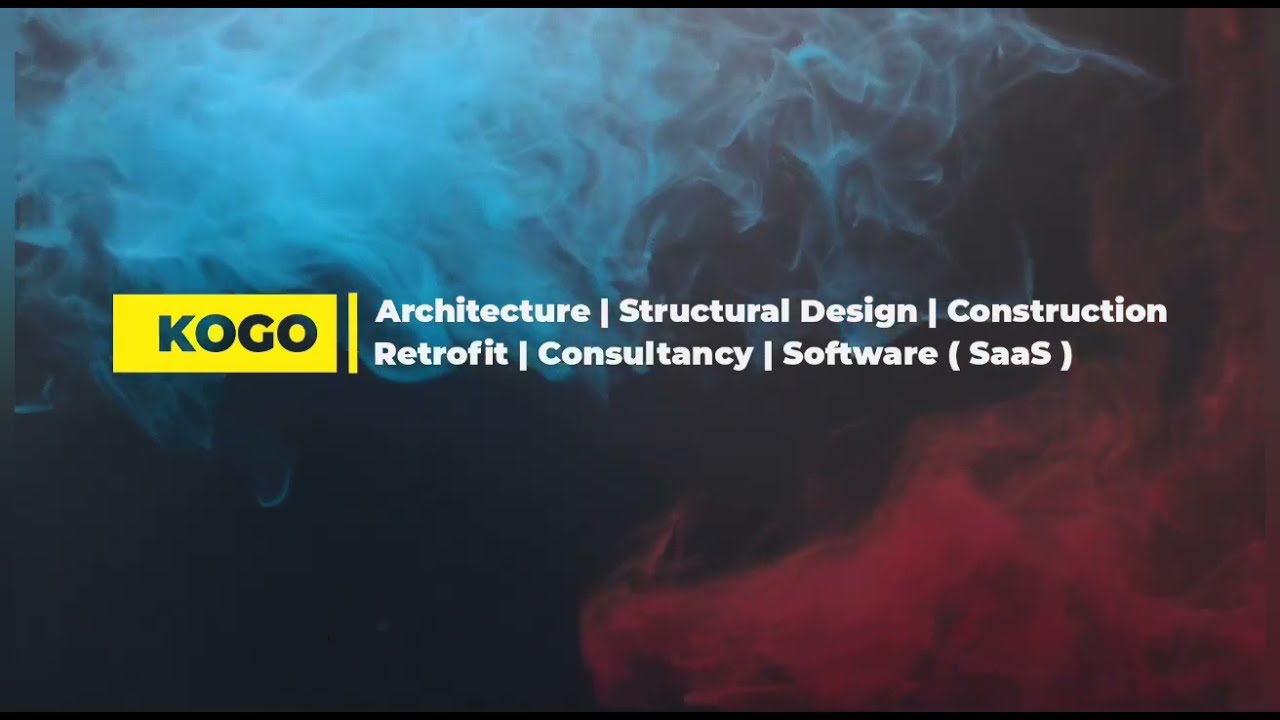The image features a vibrant, smoky background with blue mist flowing from the top left and red mist accumulating at the bottom right. The background gradually transitions from heavy black on the left to the colorful smoke mix. Within this dynamic scene, a yellow landscape-oriented rectangle stands out on the left side. The rectangle contains the word "COGO" carved out, revealing the smoky blue background through the letters. Adjacent to the word, in white font, are two rows of phrases separated by thin vertical bars: "Architecture | Structural Design | Construction" on the top row, and "Retrofit | Consultancy | Software (S-A-A-S)" below. Thin black lines border the top and bottom of the image, framing the design.